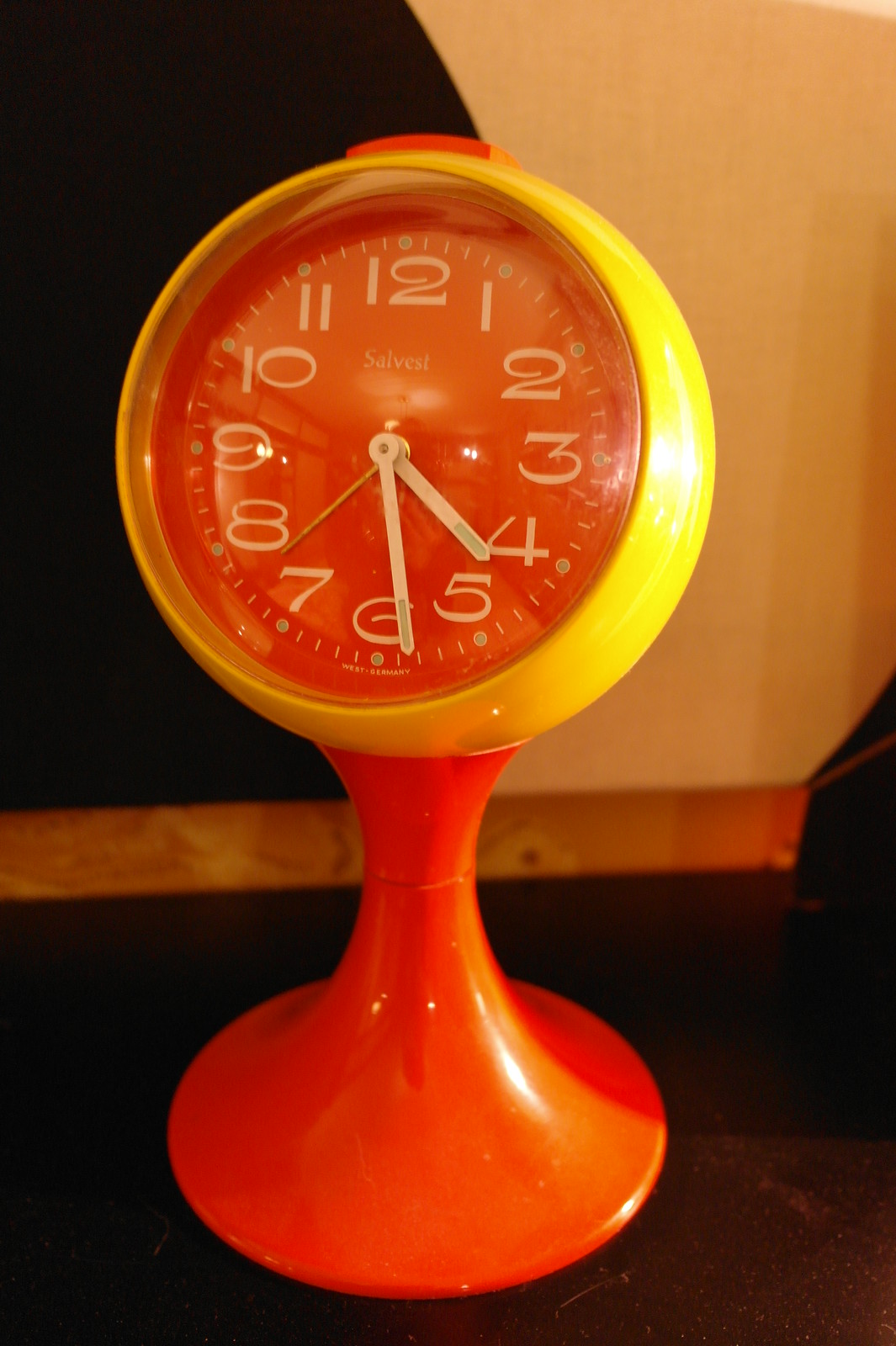This photograph features a distinctive tabletop clock with a curved, cone-shaped stand that evokes the shape of a blow horn or hourglass. The base of the stand is a large, circular disk that quickly tapers inward and then flares back outward as it ascends, connecting to the circular clock face. The clock face is framed by a yellow ring and encased in a clear plastic covering, providing a glossy, translucent surface. The face itself is a striking orange or potentially red hue, adorned with stylized white numbers and white hands for the hours and minutes, alongside a thinner gold second hand. The brand name "Salvestre" is prominently displayed at the top of the clock face. Sitting on a dark, flat surface, the clock's backdrop reveals a tan and black wall with brown trim at the bottom, indicating it is placed on a wooden or similar tabletop surface. Additionally, a large red button is visible on top of the clock, enhancing its functional and design aesthetic.